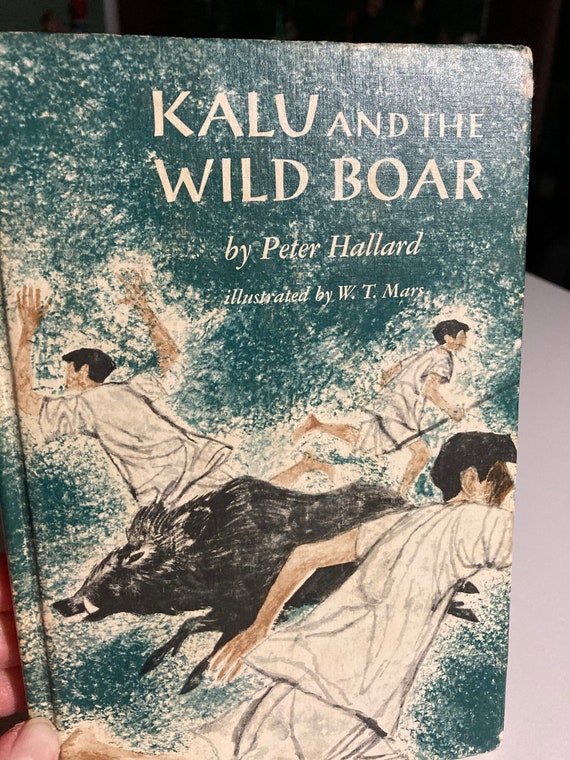The photograph features an old, worn book with a faded cover titled "Kalu and the Wild Boar" by Peter Hallard, illustrated by W.T. Mars. The book is held by a person whose white-skinned hand, with the thumb's fingernail visible, is located in the bottom left corner of the image. The background consists of a very dark upper section extending from the top left to the top right corner and a creamy-colored bottom right section, suggesting harsh lighting that implies the image was taken at night. The cover illustration, predominantly green with some cream accents, depicts three young boys with light skin and dark black hair, all dressed in white shirts and shorts, and barefoot. One boy in the top right corner wields a spear, while another figure runs in the left direction. The wild boar, with brown hair and a notable white mark around its nose and mouth, charges leftward.